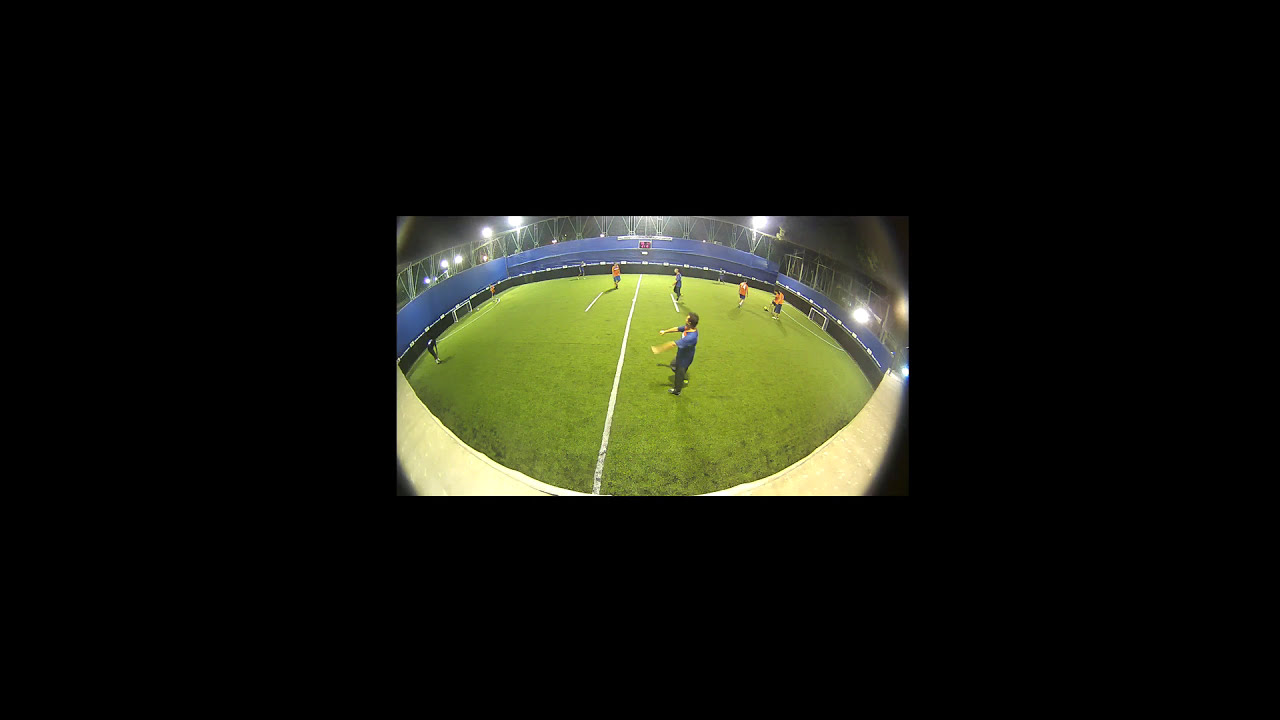The image depicts an enclosed soccer field with short, light green grass, giving it an indoor-like appearance despite the possibility of it being outdoors. The field is surrounded by a tall blue tarp that acts as a barrier, with a smaller dark blue fence featuring white railings nearby. The field is illuminated by numerous spotlights and includes a grid-style structure overhead. A black and white scoreboard with red LED lights is positioned centrally on the fencing. Players are actively engaged in a game, with around four to five players in orange and black uniforms and a similar or slightly fewer number in blue uniforms. There are two goals, one at each end of the field, demarcated by white lines and additional markings around the goal areas.